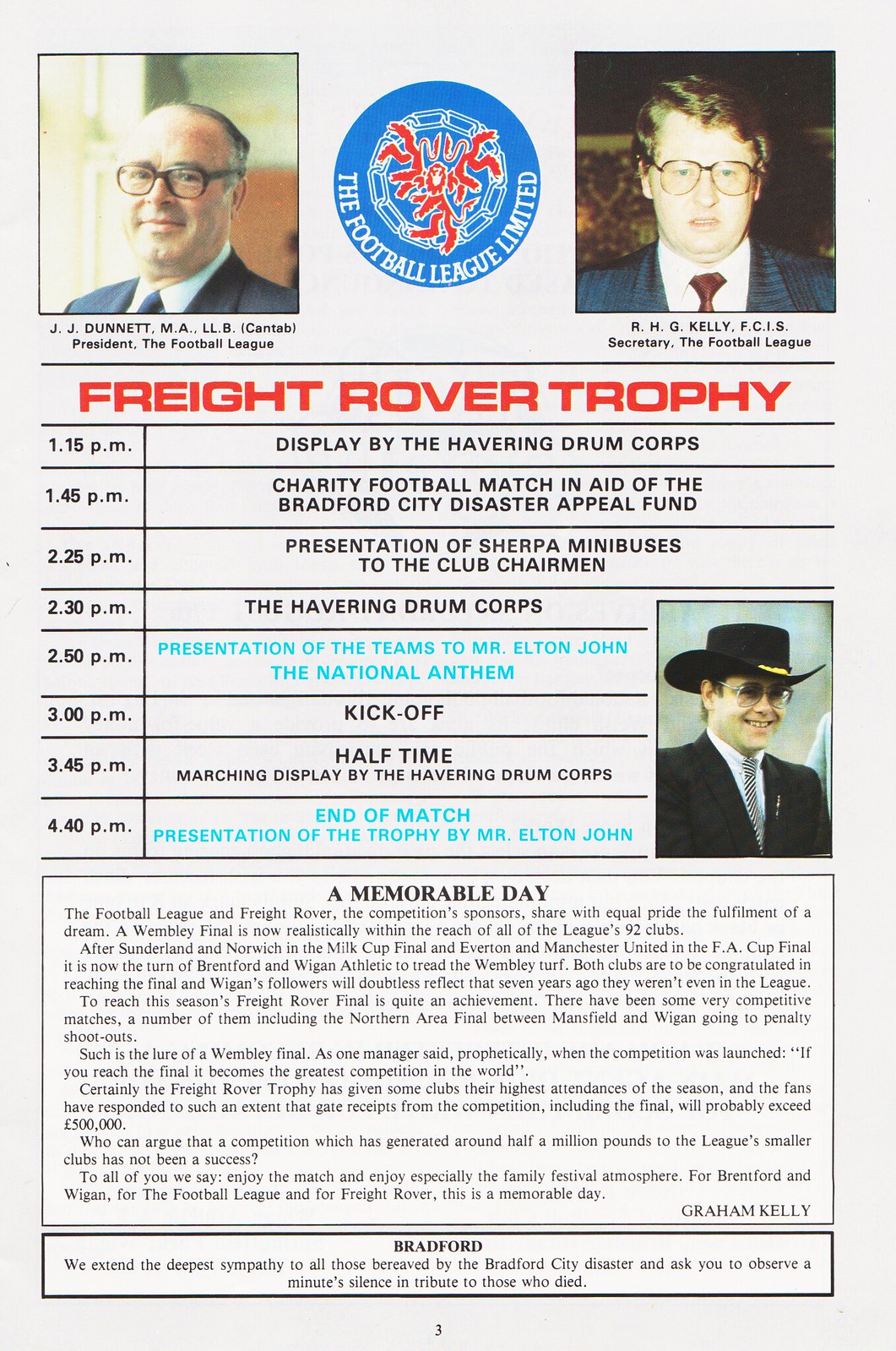This image depicts a tall, rectangular page from a magazine or advertisement with a light, off-white background, marked as page three. Dominating the top center is a blue circle featuring a logo of a red illustration encircled by a blue chain, accompanied by the curved white text, "The Football League Limited." Flanking the logo are two photographs: to the left, an older man with glasses identified as J.J. Dunnett, M.A., L.L.B. (Cantab), President of the Football League; and to the right, a younger man with glasses named R.H.G. Kelly, F.C.I.S., Secretary of the Football League. Below these images, in striking red font, is the title "Freight Rover Trophy." The page further details various scheduled events, such as a Display by the Havering Drum Corps at 1:15 p.m., a Charity Football Match at 1:45 p.m. in aid of the Bradford City Disaster Appeal Fund, the presentation of Sherpa minibuses to the club chairman at 2:30 p.m., followed by a kickoff at 3:00 p.m. and halftime activities at 3:45 p.m. Each event is meticulously timed, creating an organized and informative timeline.